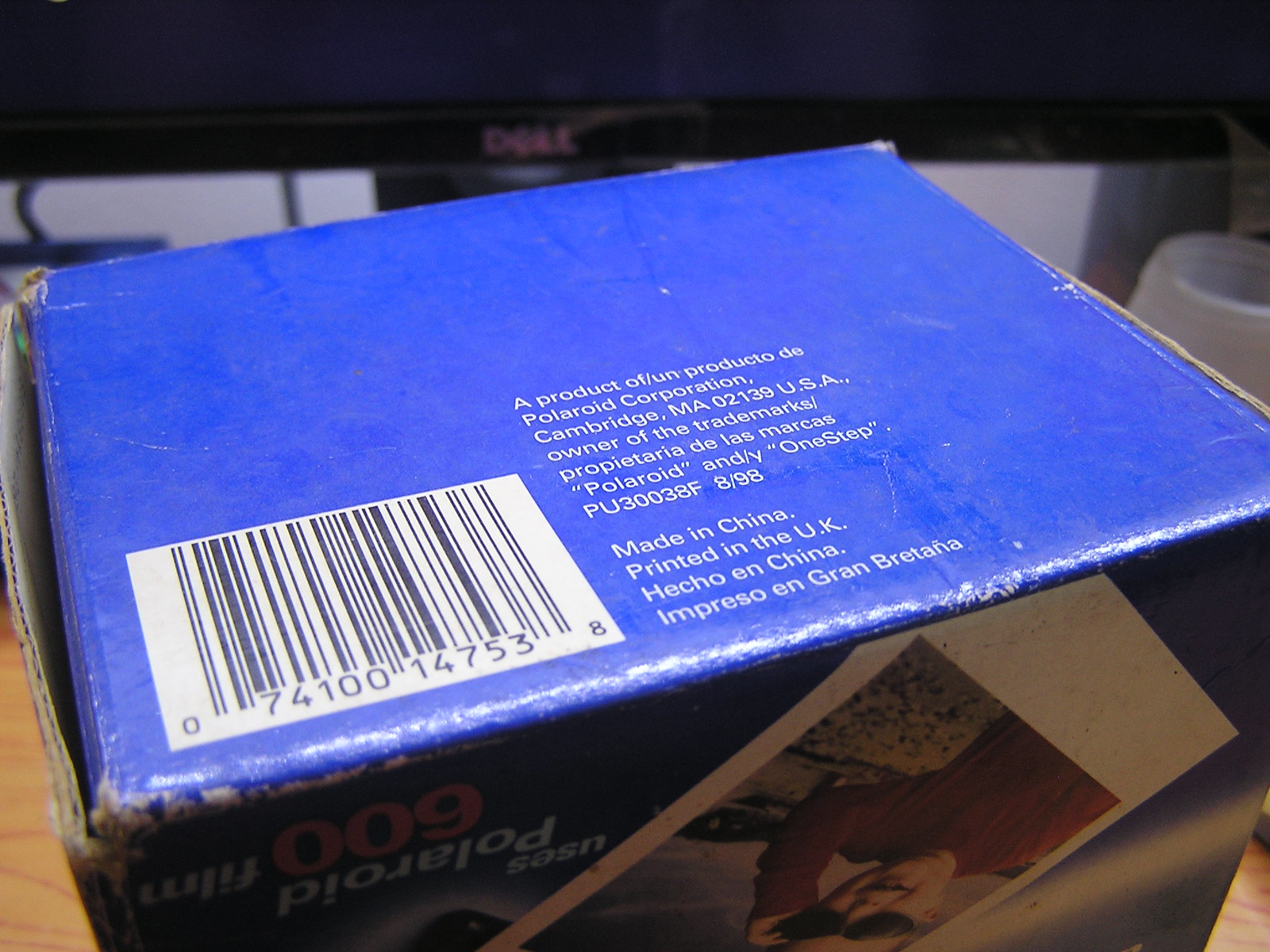The photograph captures the bottom side of a Polaroid film package, specifically a Polaroid 600 film box. The packaging is made of blue cardboard and prominently features a white bar containing a black-printed UPC code. On the visible side of the box, which is oriented upside-down, there is an image of a Polaroid picture along with text that reads "Polaroid 600 film." The bottom of the package is printed with details indicating the product's origin: "A product of Polaroid Corporation, Cambridge, Massachusetts 02139, USA," along with a statement that the Polaroid Corporation owns the associated trademarks.